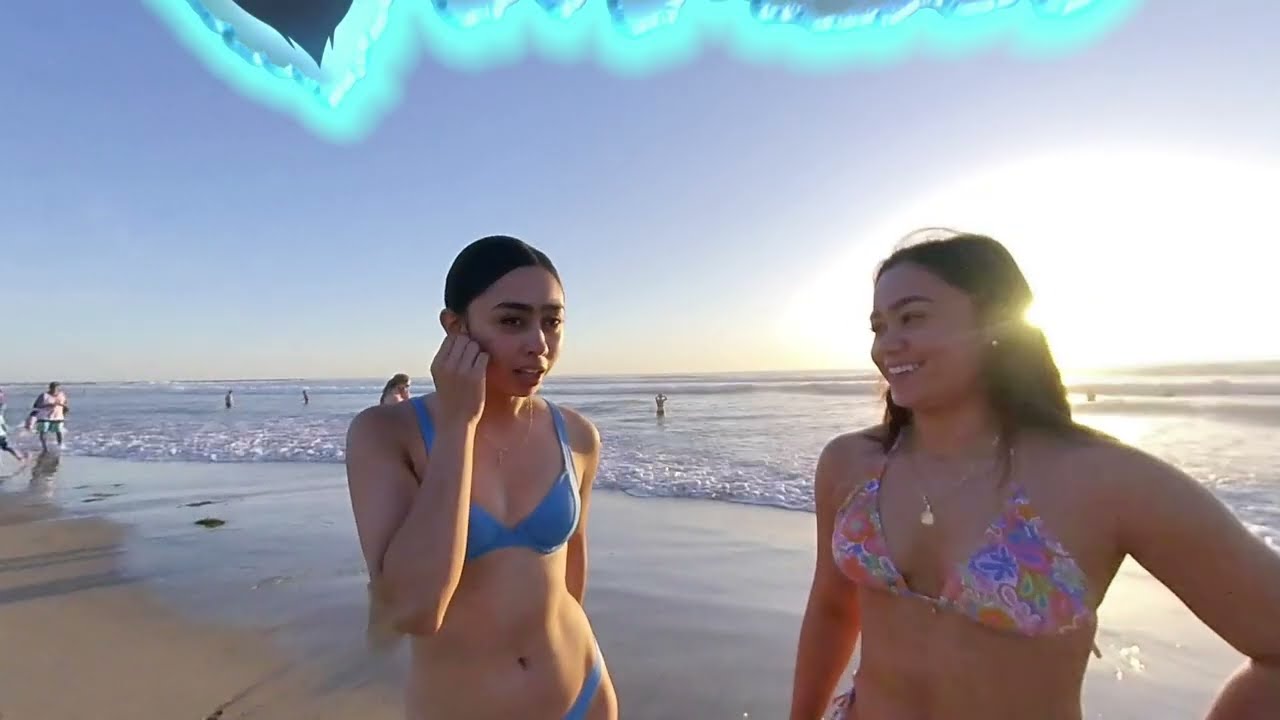In this vibrant beach scene, two young women stand side by side in the foreground. The woman on the left, with dark hair and donning a light blue bikini, has her right hand to her ear, possibly trying to clear water from it. Her friend, also with long dark hair, stands to her right wearing a brightly colored floral print bikini top and is smiling warmly at her. The sandy beach forms their base, and behind them, the tide line and surf of the ocean can be seen, along with several people either walking along the shore or playing in the foamy waves. The sky overhead is a clear blue with the sun lowering towards the horizon, casting a golden hue across the scene, indicating that it's approaching sunset. At the very top of the image, a bright turquoise distortion, resembling a vivid blue rip, adds a unique touch to the photograph.